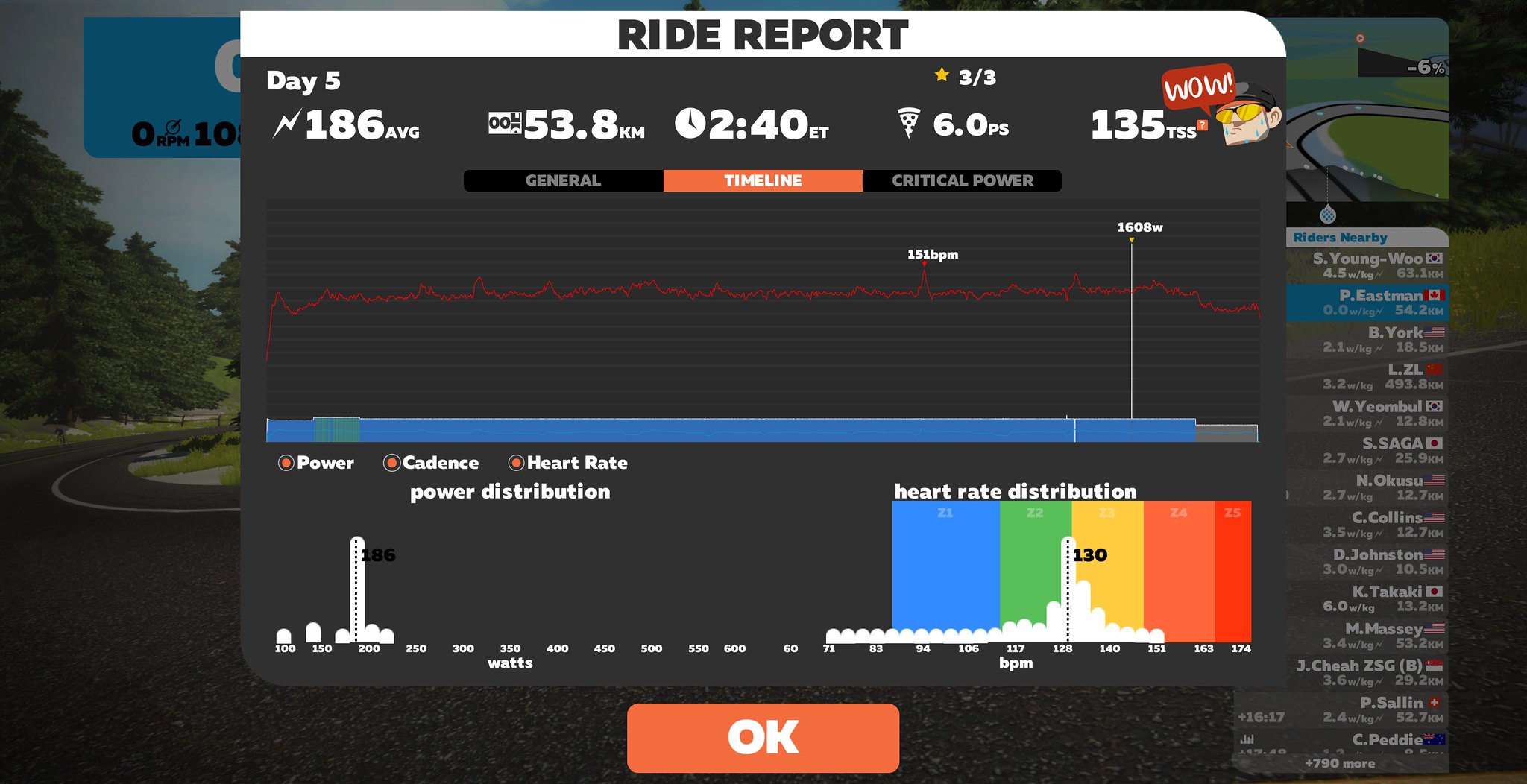The image depicts a detailed fitness app screenshot, likely from a virtual reality biking exercise. The background features a blackish-gray hue, with a white strip at the top displaying "Ride Report" in black letters, followed by "Day 5." Below this, the screen provides specific data: an average heart rate of 186 bpm, a distance of 83.8 kilometers, and a timestamp of 2:40 PM Eastern Time. The interface includes two primary graphs: one illustrating the power distribution in watts and the other showing the heart rate distribution in beats per minute (BPM) with vibrant colors. Additionally, the layout features the names and statistics of various individuals on the left. At the bottom, there's an orange rectangle with a white "OK" button, signaling the end of the report.